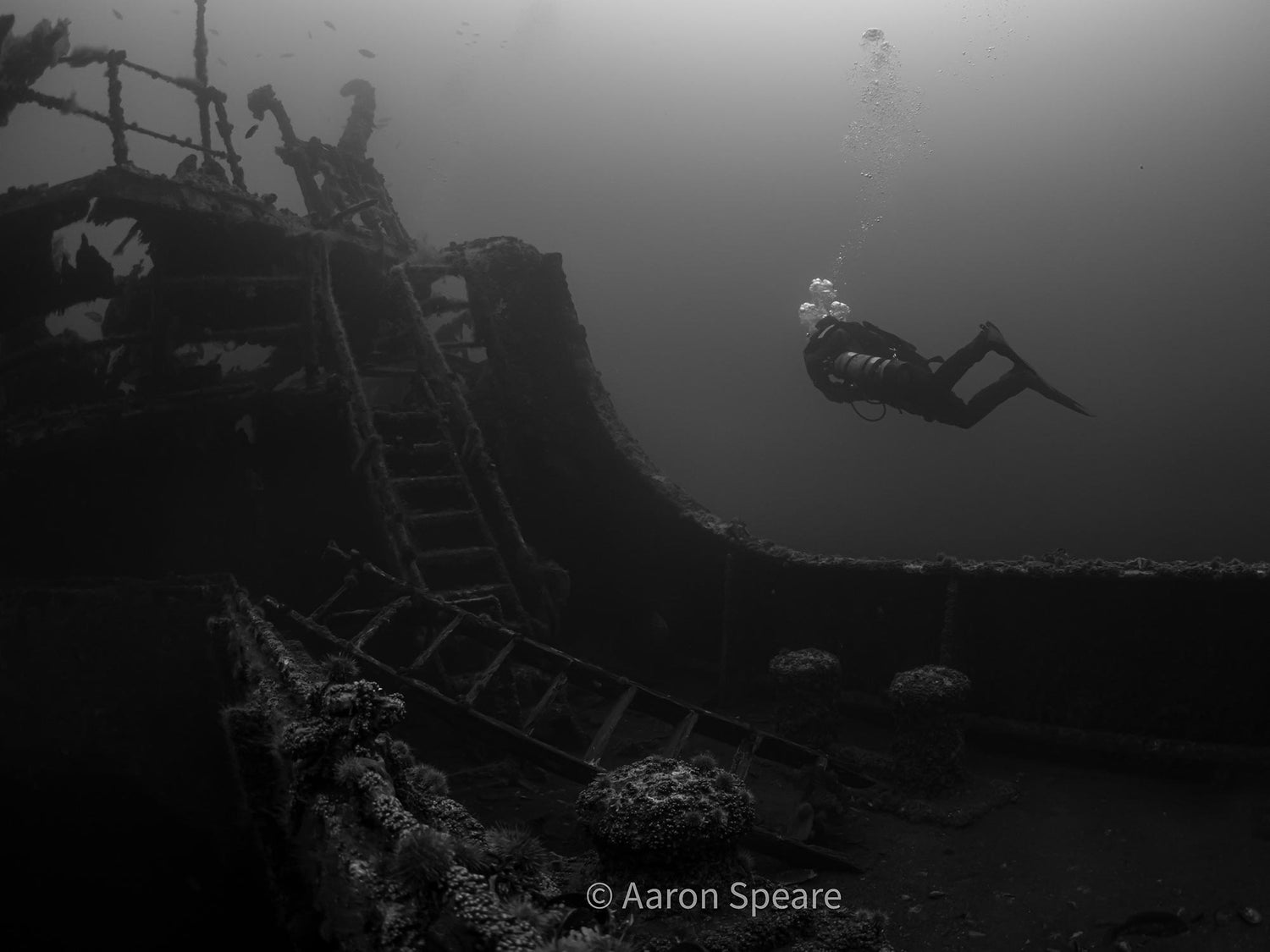The monochromatic underwater photograph depicts a scuba diver exploring a haunting shipwreck. The diver, equipped with an oxygen tank and flippers, releases large bubbles as they swim parallel to the wreck. The ship, an ancient and corroded relic, is shrouded in sea plants and coral that encrust the railings, ladders, and various other parts of the broken vessel. Ladders, both fallen and intact, punctuate the scene, which is visually divided into a dark, unsettling underwater expanse and a lighter, almost ethereal surface where natural light filters through. The entire composition carries a sense of eerie stillness, accentuated by the dark gray tones of the water juxtaposed against the faint glow from above. The photograph, marked with a copyright symbol reading "© Aaron Speare," evokes an unsettling, almost ghostly feeling, as it captures the frozen desolation of the submerged ship.